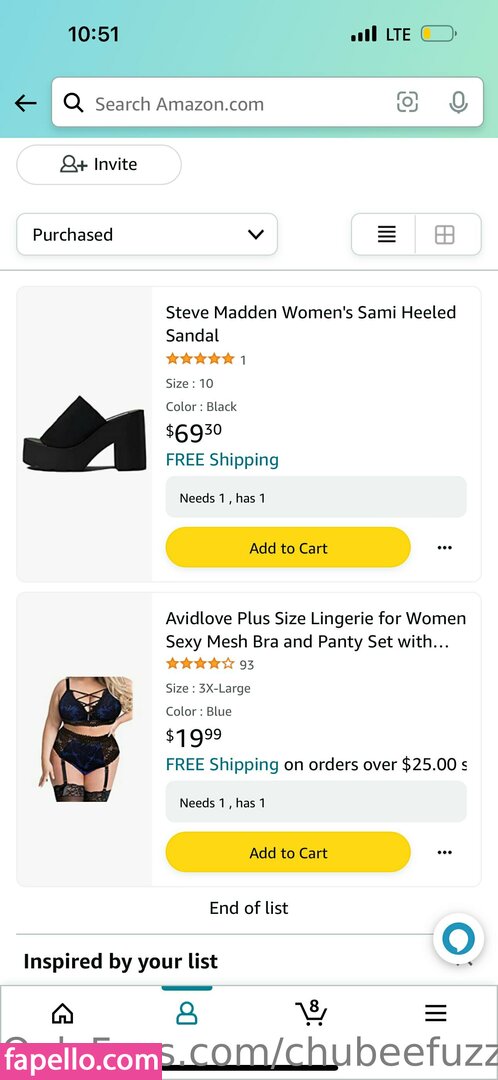The screen displays a smartphone interface at 10:51 AM with approximately 20% battery life remaining. At the top, a search bar is prominently visible with the text "search amazon.com." Beside the search bar is an "Invite" button featuring a generic person icon with a plus sign.

Below the search bar, a dropdown menu labeled "purchased" is visible. Directly beneath this menu, an image of a black shoe appears with the description "Steve Madden Women's Semi-heeled Sandal." The shoe has received five stars from one review, is available in size 10, and is priced at $69.30 with free shipping. A yellow "Add to Cart" button is situated below the shoe details.

Further down the screen, another product is listed: "Avidlove Plus Size Lingerie for Women Mesh Bra and Panties Set." This item has garnered four out of five stars from 93 reviews, is available in size 3X Large, and comes in the color blue. The pricing for the lingerie set is $19.99, with free shipping on orders over $25.